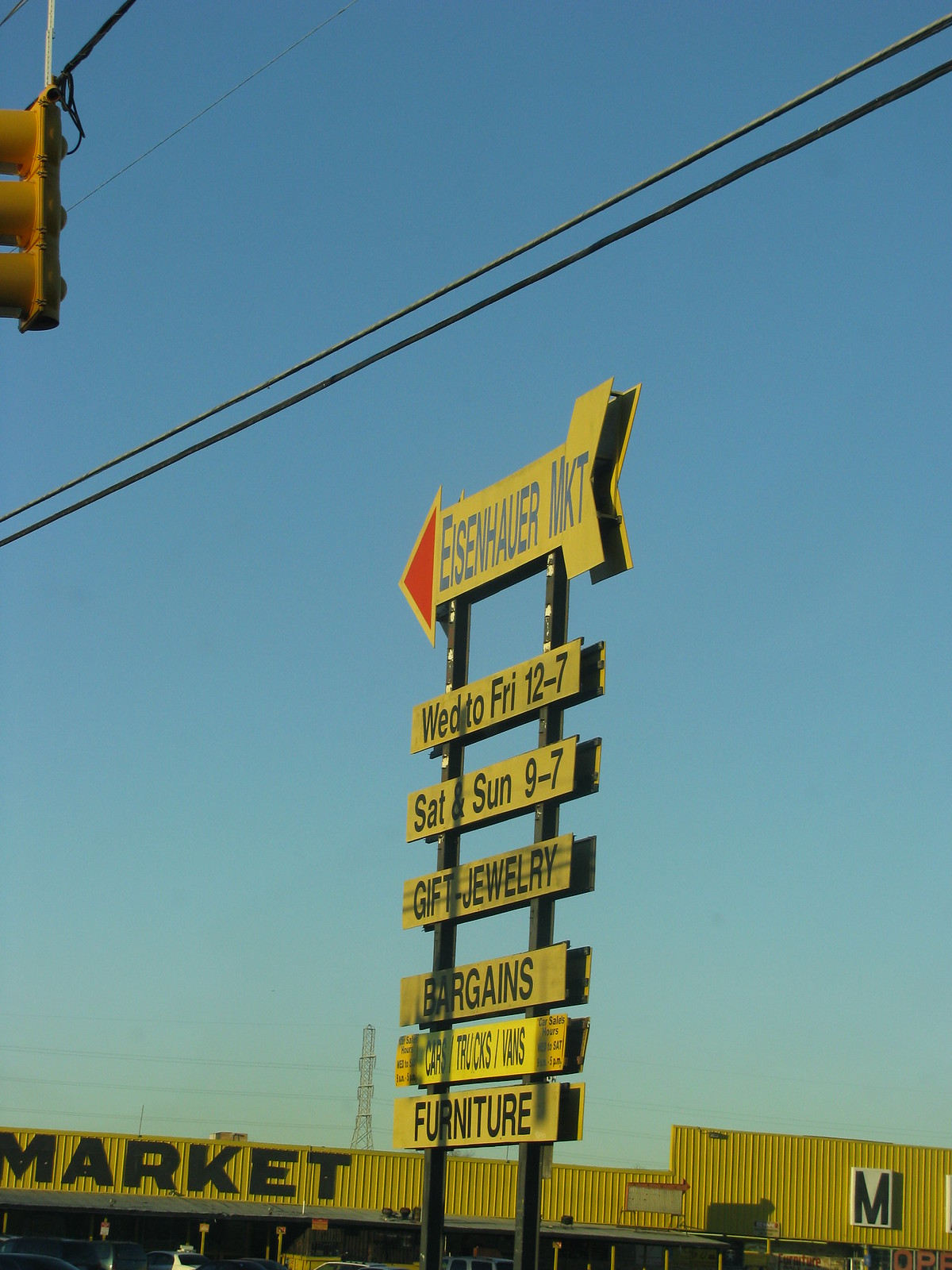This outdoor color photograph features a prominent market sign set against a backdrop of a light blue sky. At the bottom of the image, the yellow rooftop of a flat-roofed building is visible, with the word "market" inscribed in black letters on the left side. 

In the foreground, there are two rectangular black poles extending upwards into the midsection of the photograph, supporting a series of signs. The topmost sign is a yellow arrow with a red tip, displaying "Eisenhower Market." Below this arrow, several smaller horizontally-mounted signs follow, each with a yellow background and black letters. The text on these signs includes operating hours: "Wednesday to Friday, 12 to 7," and "Saturday and Sunday, 9 to 7," followed by categories of items available such as "Gift Jewelry," "Bargains," and "Furniture." There is also a partially obscured sign that is difficult to read and another sign featuring "Cars, Trucks, Vans."

Additionally, a traffic signal light can be seen hanging in the upper left corner of the image, contributing to the lively market atmosphere.